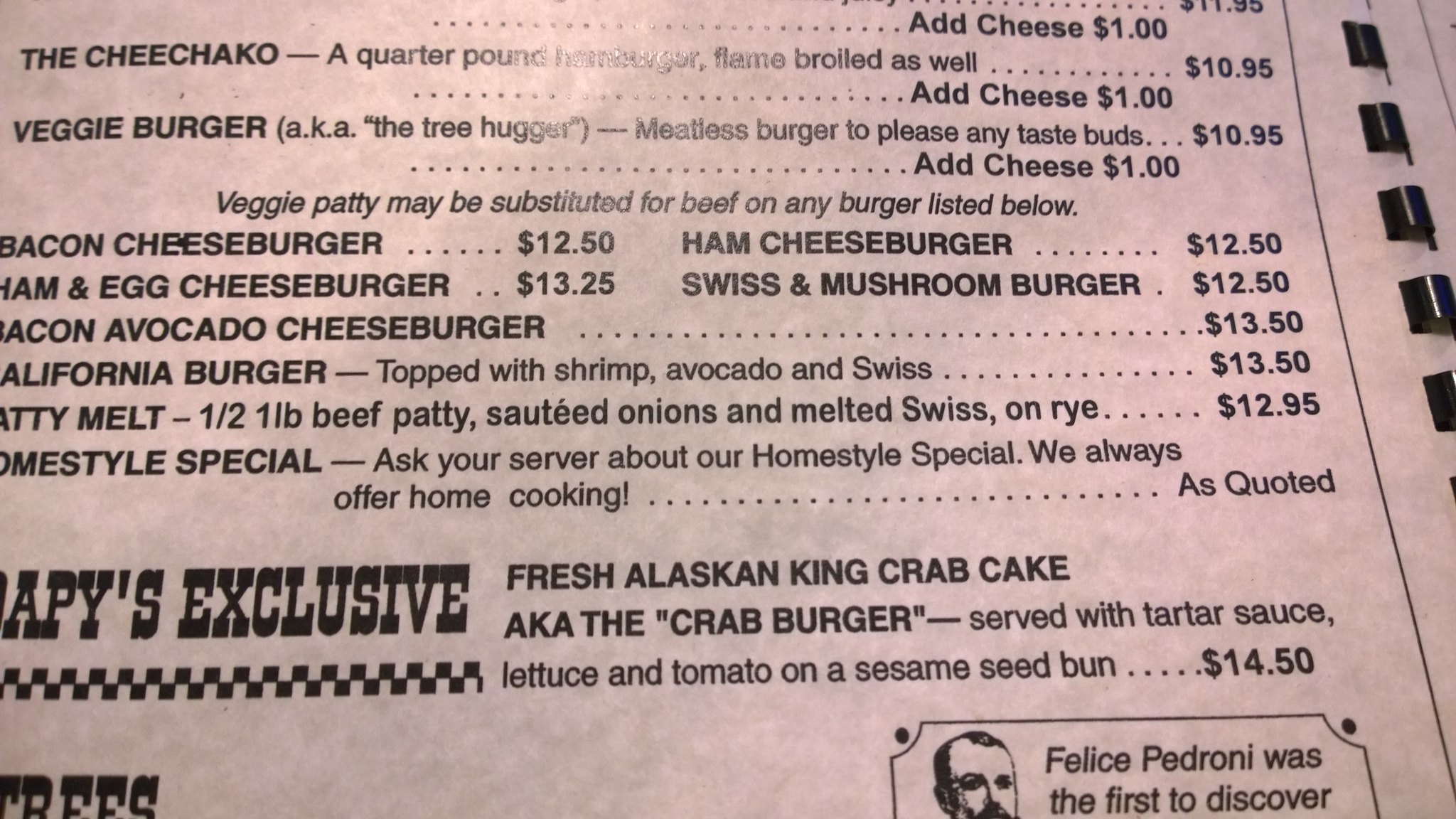Close-up of a section of an old-fashioned styled menu bound with a unique plastic coil, which uses individual plastic rings to hold perforated pages together. The menu features a rustic aesthetic, with a background reminiscent of aged parchment paper and text in an Old West-style font.

At the bottom right, a decorative border encloses the partial text, "Felice Pedroni was the first to discover," next to a sketch in the style of the late 1800s or early 1900s, hinting at historical significance. The visible sections of the menu list several gourmet burger options and their prices:

- **Exclusive Fresh Alaskan King Crab Cake (The Crab Burger):** Served with tartar sauce, lettuce, and tomato on a sesame seed bun for $14.50.
- **Chief Choco (CHEECH):** A quarter-pound flame-broiled burger for $10.95, with an option to add cheese for $1.
- **Veggie Burger (The Tree Hugger):** A meatless burger for $10.95, with an option to add cheese for $1. The veggie patty can be substituted for beef on any other burger.
- **Bacon Cheeseburger:** $12.50
- **Ham Cheeseburger:** $12.50
- **Ham and Egg Cheeseburger:** $13.25
- **Swiss and Mushroom Burger:** $12.50
- **Bacon Avocado Cheeseburger:** $13.50
- **California Burger:** Topped with shrimp, avocado, and Swiss cheese for $13.50.
- **Patty Melt:** Half-pound beef patty with sautéed onions and melted Swiss cheese on rye for $12.95.
- **Home Style Special:** Daily home-cooked special, details provided by the server.

Although some text on the left side of the menu is cropped, enough context is given to accurately infer the full names of these items.